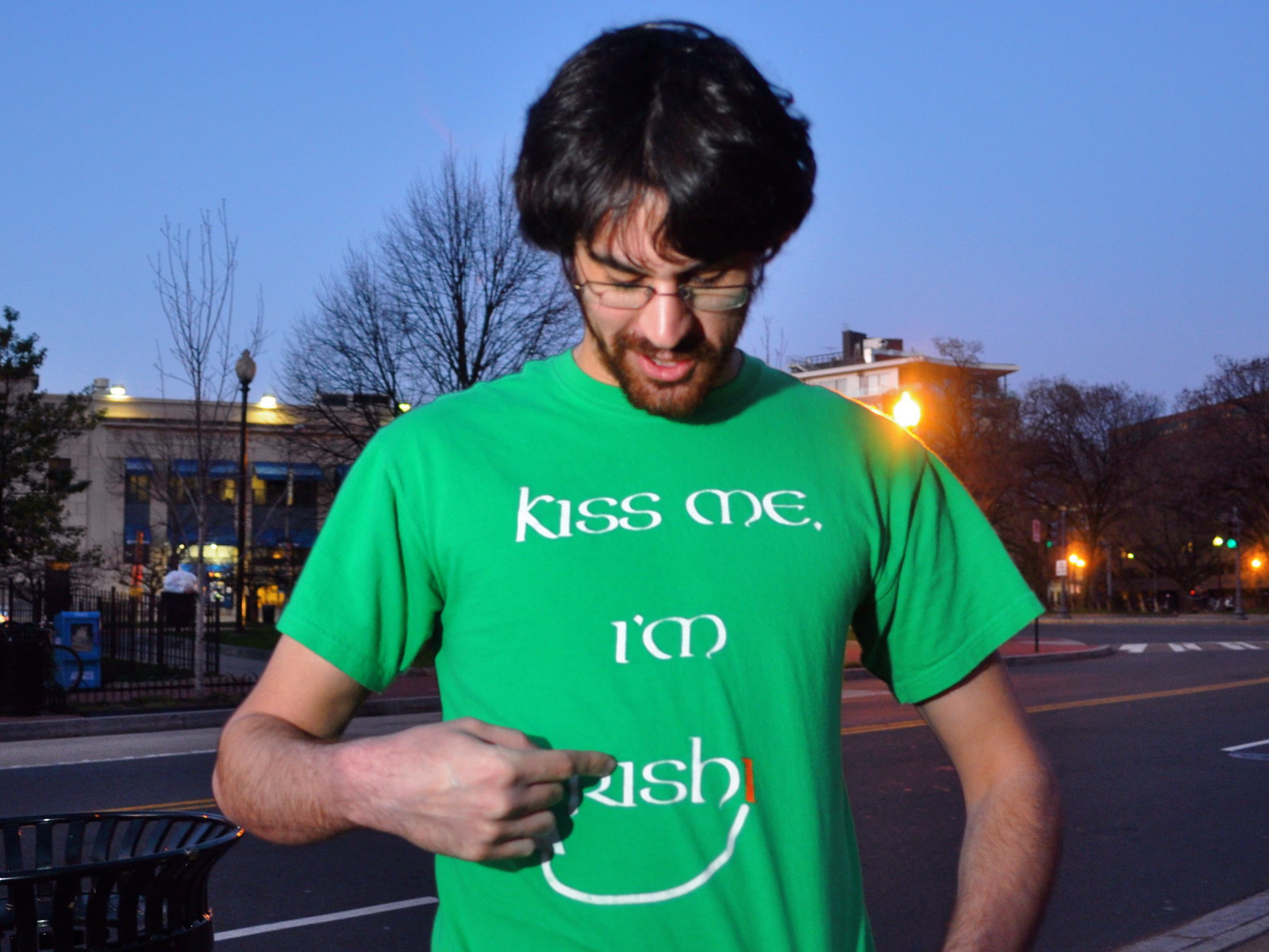In the image, a man with short black hair, glasses, and a short beard is standing in the foreground, centered and pointing to the white text on his bright green, short-sleeved t-shirt which reads, "Kiss me, I'm Irish." He has peach skin and is looking down at the text on his shirt, pointing with his right hand. The scene appears to be outdoors, likely in the evening around 7 p.m., indicated by the overall lighting and presence of illuminated streetlights. 

In the bottom left corner behind the man, the corner of a trash can can be seen. The setting includes a gray road with visible yellow and white lines in the bottom third of the image. The middle third features various structures and natural elements: a tan building with some blue accents is situated to the left over his right shoulder, flanked by trees with dark green foliage to the left and right. Additional lights and another building can be seen further to the right. The top third of the image shows a light blue sky, completing the background. The colors present in the image comprise green, blue, brown, gray, purple, and yellow, adding depth and context to the evening scene.